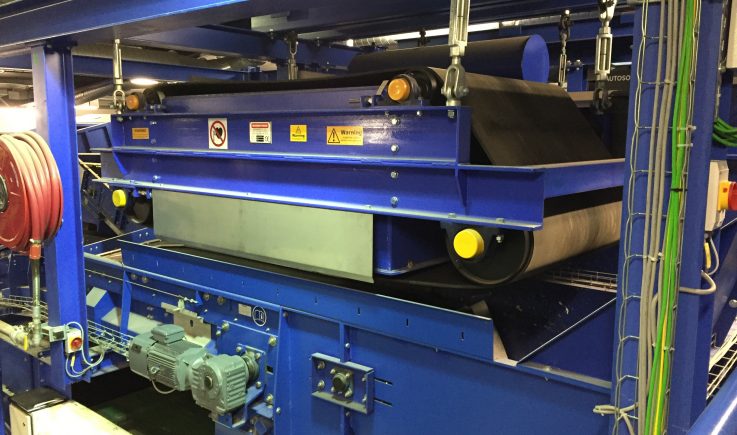This is a detailed photo of a complex industrial printing machine located in a factory. The machine is substantial in size, painted a bright blue, and constructed of metal. It prominently features a large roller wheel with a white sheet, suggesting it might be used for pressing or feeding materials through it. The machine is intricately designed with numerous screws, divots, and wires. Notable wires, colored green and gray, run up the side of the machine, indicating a network of connected systems. At the base, there are circular dials in a mint green color, likely integral components of the machine. A striking red stop button and a yellow and red button are situated on the right side. Additionally, a red coiled hose is attached to a hose stand on the right, while blue metal beams span across the ceiling above. The machine appears to be supported by four bars descending from above, adding to its structural complexity.